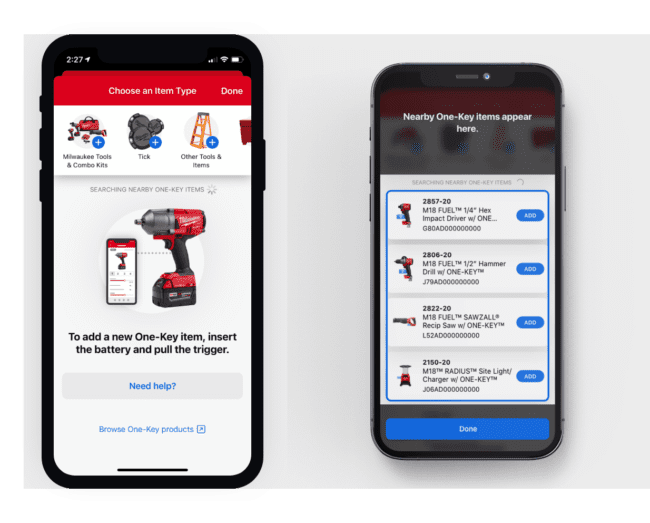The image showcases two different cell phones with various tool-related applications displayed on their screens.

On the left cell phone, which has a black frame, the time at the top left corner reads 2:27. Adjacent to this, a nearly full battery icon is displayed in white. Directly below, a red box with the text "Choose an item type" is visible. To the right of the red box, the word "Done" is shown. Below this section, the text "Tools and Combo Kits" is displayed, followed by images of various tools, most of which are red and black. To the right, the word "TICK" (spelled T-I-C-K) is visible, followed by other tools and items, including an image of a ladder above this text. Below, the phrase "Searching nearby One-Key items" is seen. Further down, an image of a red and black drill with a gray drill bit is displayed, accompanied by the instruction to "Add a new One-Key item, insert the battery and pull the trigger." At the bottom, there is a prompt reading "Need Help?"

On the right cell phone, the heading at the top reads "Nearby One-Key items appear here." Below, in a long blue box, various tool items are listed. The first is a drill, followed by a hammer drill, then a Sawzall, and finally a radius site light charger. At the very bottom, the word "Done" is displayed within a blue box.